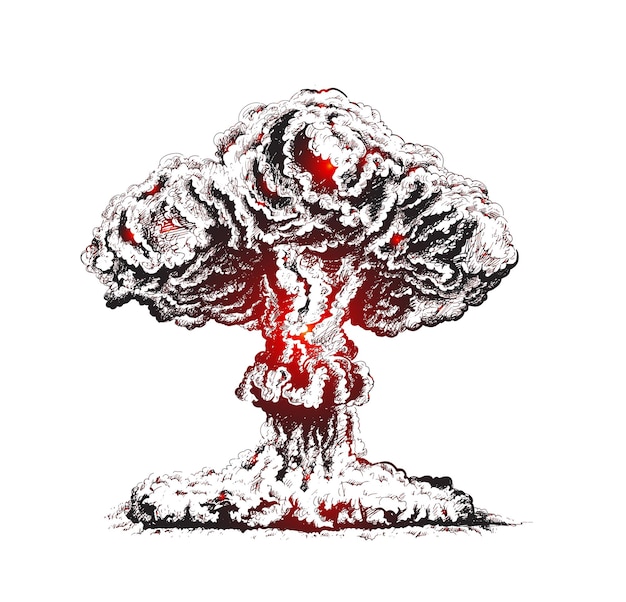This image, set against a stark white, borderless background, vividly depicts a drawing of an atomic or fusion bomb mushroom cloud. The artwork employs a monochromatic palette punctuated with shades of red. The stem of the mushroom cloud predominantly features red and white hues, suggestive of intense heat emanating from within. In contrast, the mushroom cap, intricate with folds and convolutions, is rendered primarily in black and white, with slivers of red emerging through the fissures, especially concentrated at the upper sections. The explosive form, deviating from the traditional singular plume, resembles multiple overlapping heads of cabbage or lettuce. These enveloping shapes further enhance its abstract nature. Without any text accompaniment, the artwork remains an evocative piece, blending the raw power of an explosion with an abstract, almost organic form.